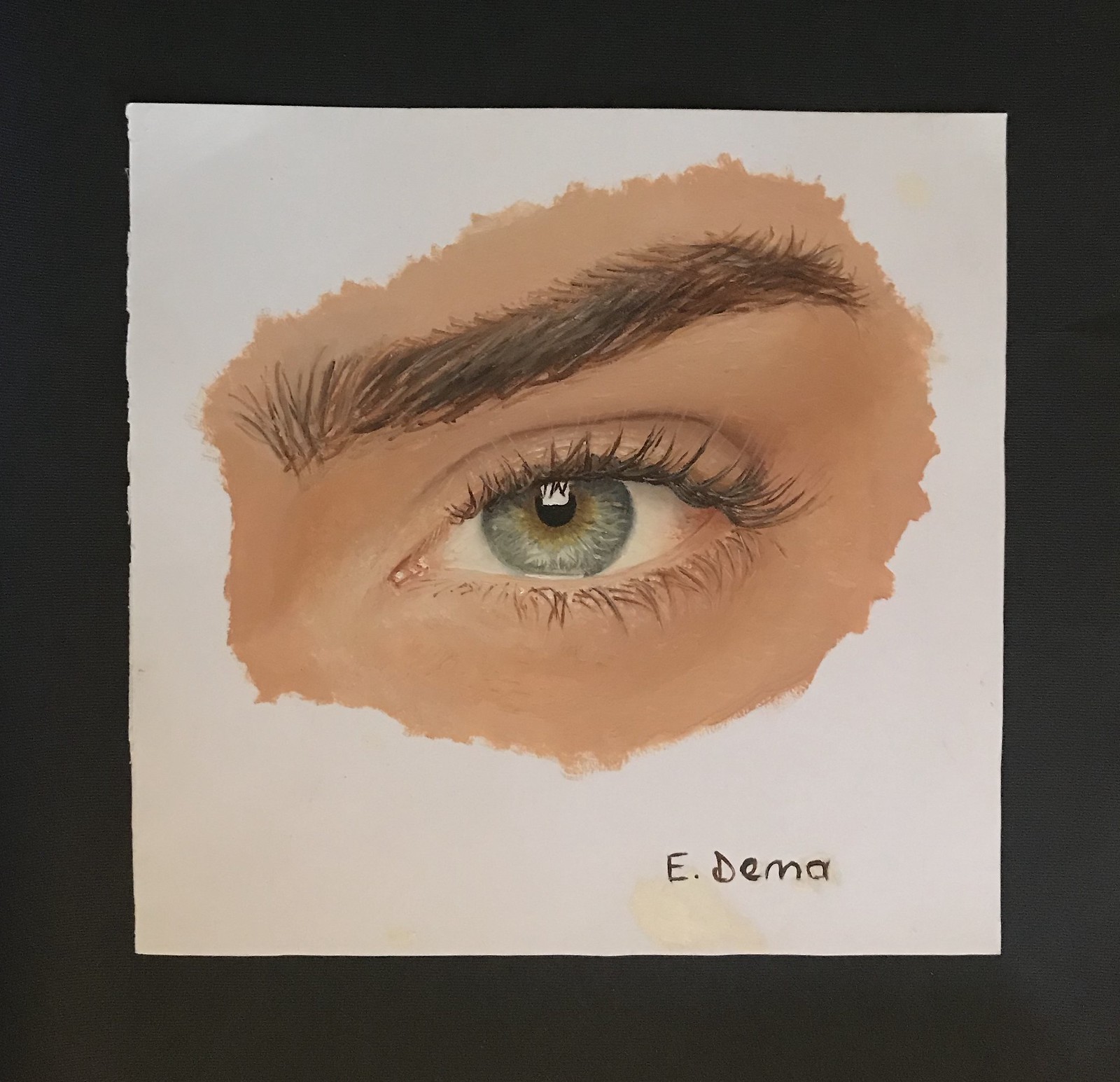The image depicts a meticulously painted or drawn eye framed by a bold, black border, with an off-white to gray background. The central focus is the eye, accompanied by the surrounding skin area above the eyebrow. The person appears to have Caucasian skin. The eyebrow is prominently featured, made up of thick, almost black hairs that might even appear grayish in some light. The eye itself is striking, with long, dark eyelashes both on the upper and lower lids. The iris is a captivating mix of dark blue to grayish-blue hues, surrounding a jet black pupil that features a small, rectangular highlight reflecting light. The artwork captures the intricate details of the eye region, bordered by a cloud-like shape emphasizing the eye's outline. Toward the bottom right corner of the piece, the name "E.Dema" is clearly inscribed.